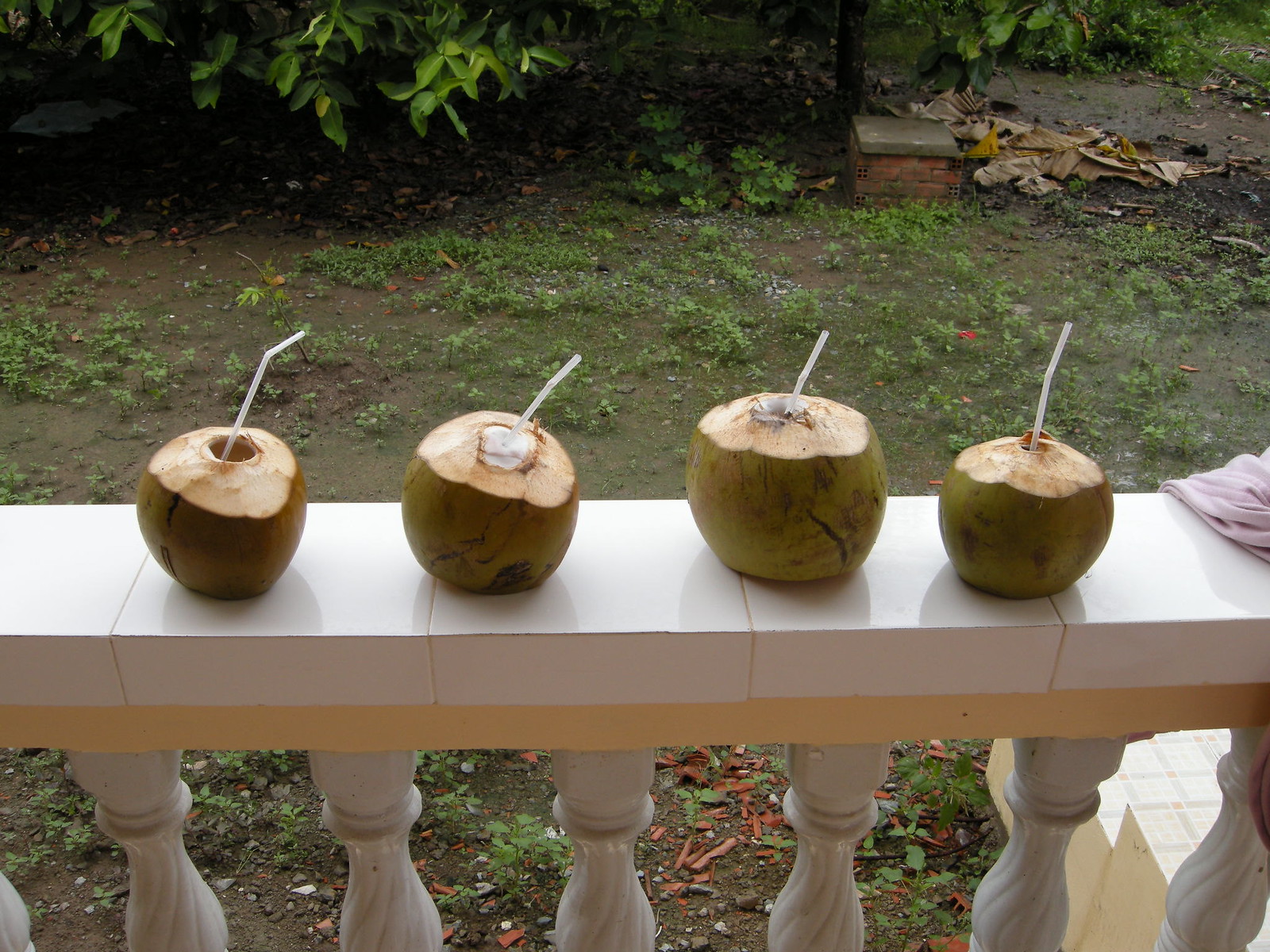The image captures a detailed scene of a porch area overlooking a backyard. Four green coconuts, each with its top cut open and a plastic bendable straw inserted, are lined up along a thick, white banister. The banister and the ornate vertical spindles supporting it are constructed from what appears to be white concrete. There is a pink fabric, possibly a sweater, draped over the banister next to the coconuts. The sizes of the coconuts vary slightly, with at least one larger than the others, and the cut tops reveal the white inner flesh of some. The scene behind the railing includes a yard that is mostly dirt with patches of grass and some debris towards the top right. A large tree or bush adds greenery in the background, enhancing the scene's natural feel. Overall, the image blends decorative elements of the porch with the rustic charm of the yard beyond.